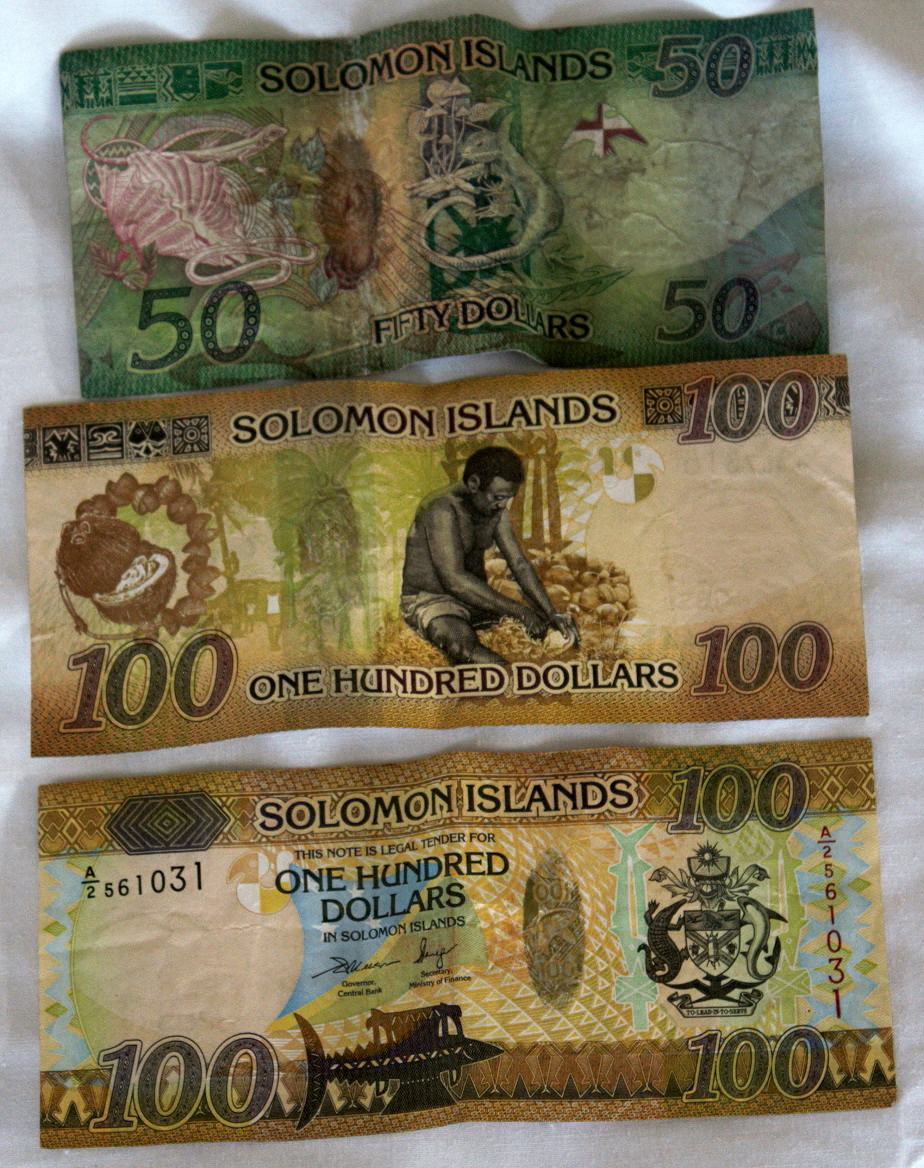The image showcases three different currency notes from the Solomon Islands, placed on a white background. The top note is a vibrant green $50 bill featuring a dominant theme of sea life, including pink clams and various sea creatures. The number 50 is prominently displayed in three corners, with the denomination $50 marked along the bottom border. The middle note is a gold-colored $100 bill. Its design includes an image of a shirtless man in shorts, seemingly engaged in the task of peeling a fruit or vegetable beside an open coconut. This note also has the number 100 in three corners and $100 across the bottom. The last bill, a blue and green $100 note, displays the reverse side of the currency. It features the Solomon Islands flag, characterized by its blue, green, and yellow stripes, and the national crest, which consists of a shield flanked by a shark on the right and an alligator on the left, along with other cultural symbols and intricate decorative elements.